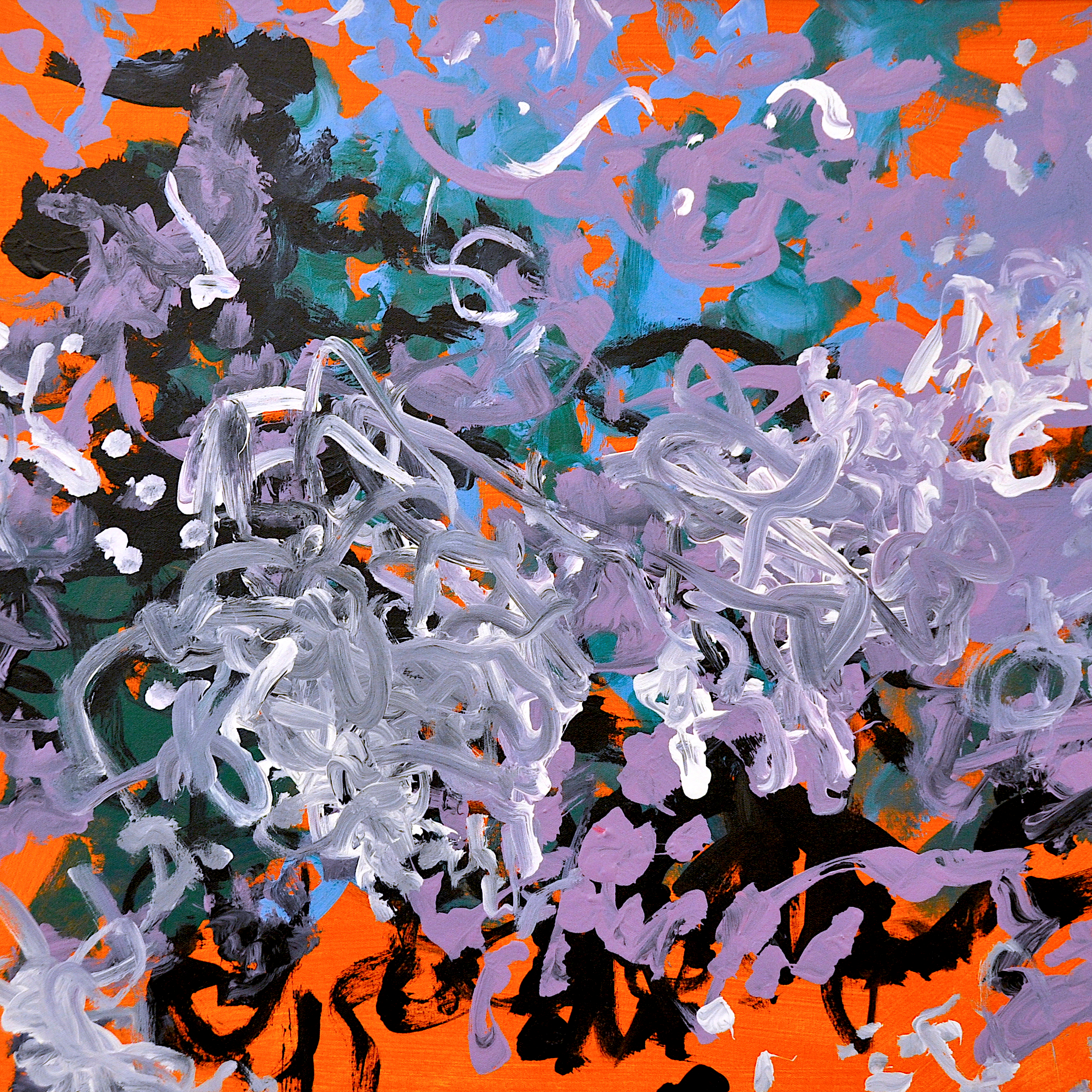This is a vibrant, abstract painting on a square canvas, characterized by its dynamic interplay of various colors and textures. The piece prominently features a bold array of colors, including black, yellow, orange, blue, purple, dark green, teal, white, and gray. The background is a coral-orange hue, which serves as a contrasting foundation for the swirling, curling, and sometimes dotted brushstrokes.

The painting is replete with movement and energy, with areas that exhibit distinct brush marks and other sections that appear almost finger-painted, adding a layered sense of texture. The brushstrokes convey a sense of disorganized whimsy, with some areas showing the canvas tooth through thinning paint. Black and dark green dominate the left-hand side of the canvas, while vibrant streaks of orange are concentrated at the bottom right. Lilac shades primarily occupy the top right, blending into thick, textured sections where violet and white hues intermingle to create grayish-black areas.

Overall, the piece is a lively mosaic of color and form, devoid of any recognizable objects or text, allowing viewers to fully immerse in its abstract complexity and vivid, emotive strokes.